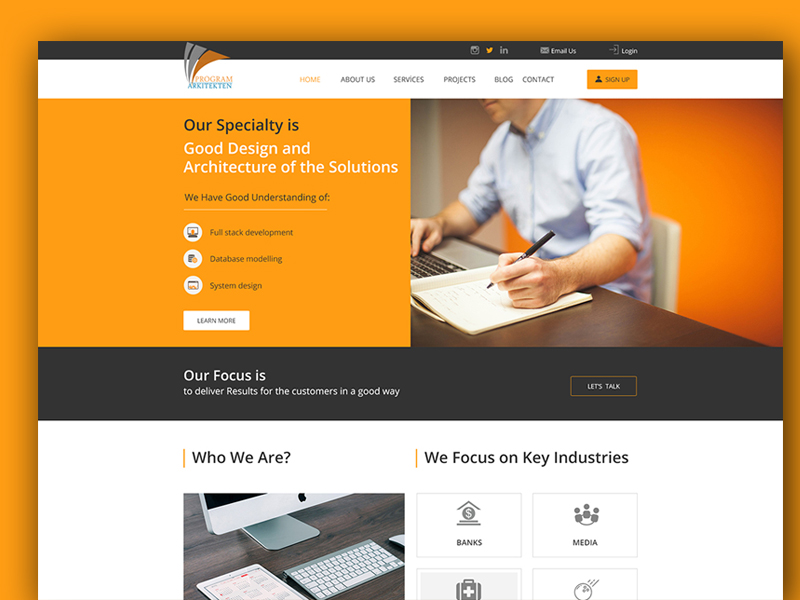This is a screenshot of the Program Architectin application. The interface prominently features a vibrant orange as the main highlight color, contrasted against a dark charcoal gray. The design employs a shadow box effect, giving the impression that the main content area is slightly elevated above the orange background.

In the upper left-hand corner, the Program Architectin logo is displayed against a white background in the header bar. The header bar contains navigational options listed in this order: Home, About Us, Services, Projects, Blog, Contact, and a Sign Up button. The 'Home' option is currently active.

Beneath the header bar, a large orange square occupies significant screen real estate, featuring the following text: "Our specialty is" in charcoal gray, followed by "Good Design and Architecture of the Solutions" in white. Additional text in charcoal gray reads, "We have Good Understanding of:" followed by a list including Full Stack Development, Database Modeling, and System Design. A button labeled "Learn More" is also present, inviting users to explore further details.